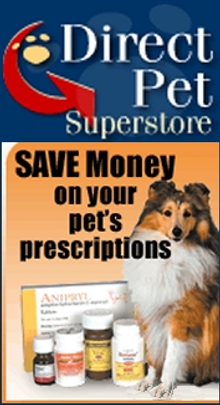In the image, the top section features a blue background with a prominent red arrow pointing down. On the arrow, the text reads "Direct Pet Superstore." Below, an orange circle contains the message "Buy Tests to Save Money on Your Pet's Prescriptions." 

In the foreground, there is a dog with striking dark ears, a darkly shaded face, black eyes, and a black nose. The dog's belly and the left side of its body are white, forming a stark contrast. The dog is standing next to what appear to be pet prescription medications, including several pill bottles. Notably, the dog's feet and the surrounding area seem poorly photoshopped, with an unnatural appearance. Additionally, the image is bordered by orange edges and overall has a low-quality feel, characteristic of an amateur advertisement.